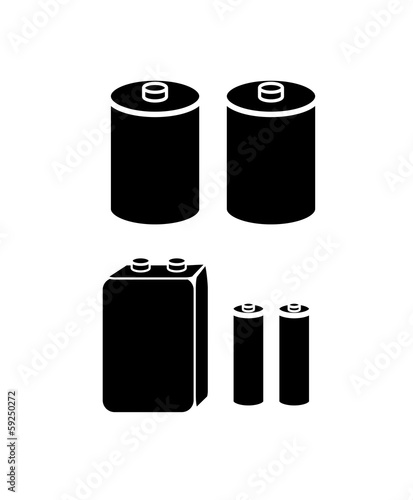The image is a black-and-white clip art illustration featuring five vertically oriented batteries on a white background. In the top left and right corners, there are two cylindrical batteries resembling C batteries, sketched in black ink with white accents to define their features, such as the positive and negative terminals. At the bottom, there are three more batteries: on the left side is a rectangular 9-volt battery with two terminals on the top, and on the right side are two identical cylindrical batteries, likely AA, featuring white outlines to distinguish various battery components. The image appears to be a stock illustration from Adobe Stock, as indicated by faint text on the side.